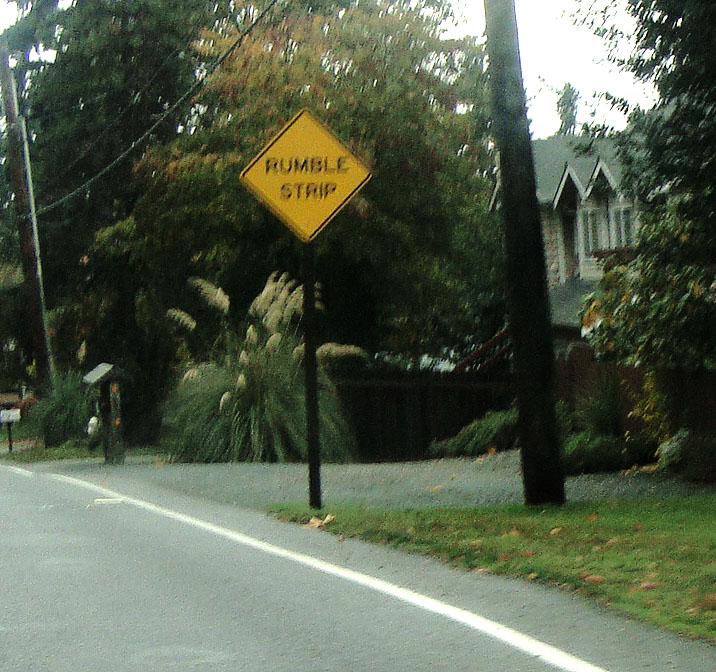The photograph captures an older, well-maintained house on the right-hand side, featuring a peaked roof and decorative upside-down V-shaped accents above the windows. The front facade appears to be adorned with stone, and there's a covered porch on the first floor. To the left, what initially seems to be a two-car garage is actually dark brown fencing, ending with tall, grassy plants exhibiting long green leaves and tall grass stalks. The house is partially obscured by numerous deciduous trees, adding a natural frame to the scene.

In the foreground, a light gray blacktop road, marked with a solid white line, leads the viewer's eye towards a prominent yellow sign. This sign, supported by a black pole, is diamond-shaped with one corner pointing upward, bearing the bold black text "RUMBLE STRIP." Adjacent to the sign stands a brown telephone pole, from which a telephone line descends and stretches across the frame, hinting at another pole on the photograph's left-hand side.